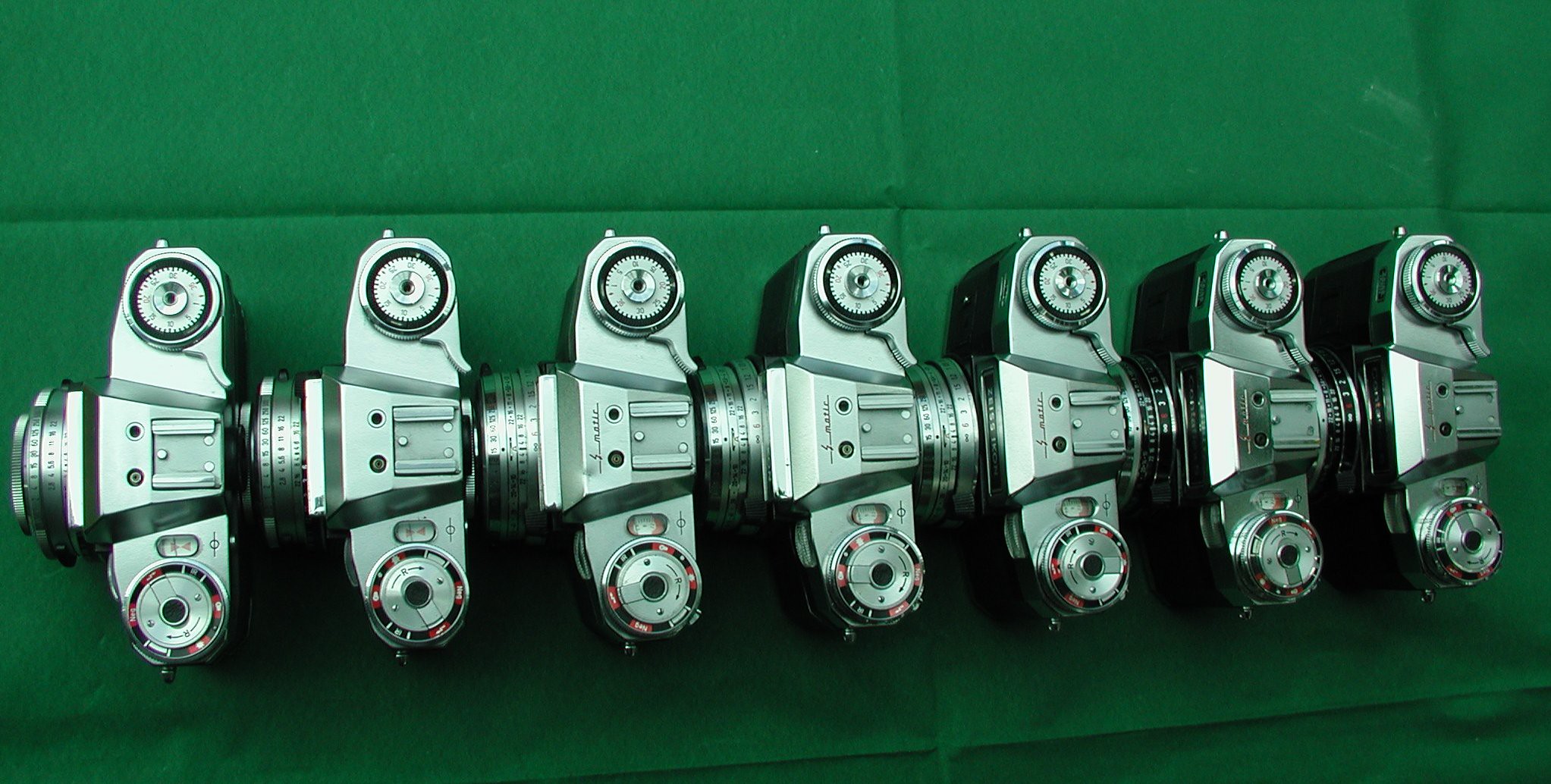In this color photograph, shot in landscape orientation, we see a meticulously arranged display of seven identical silver film cameras viewed from above. They are positioned in a tight horizontal line, each camera adjacent to the next, forming a seamless, continuous row across a dark green background that resembles a slightly darker, solid-colored paper tablecloth or tissue paper, with visible fold marks. Each camera features a distinctive circular dial and winding mechanism located on both the top and the left side of the body, while the lens, which includes a red and black band around it and intricate numbering, points to the left. The overall layout and detailed presentation of the cameras highlight their precision and uniformity, creating a visually cohesive and striking image.